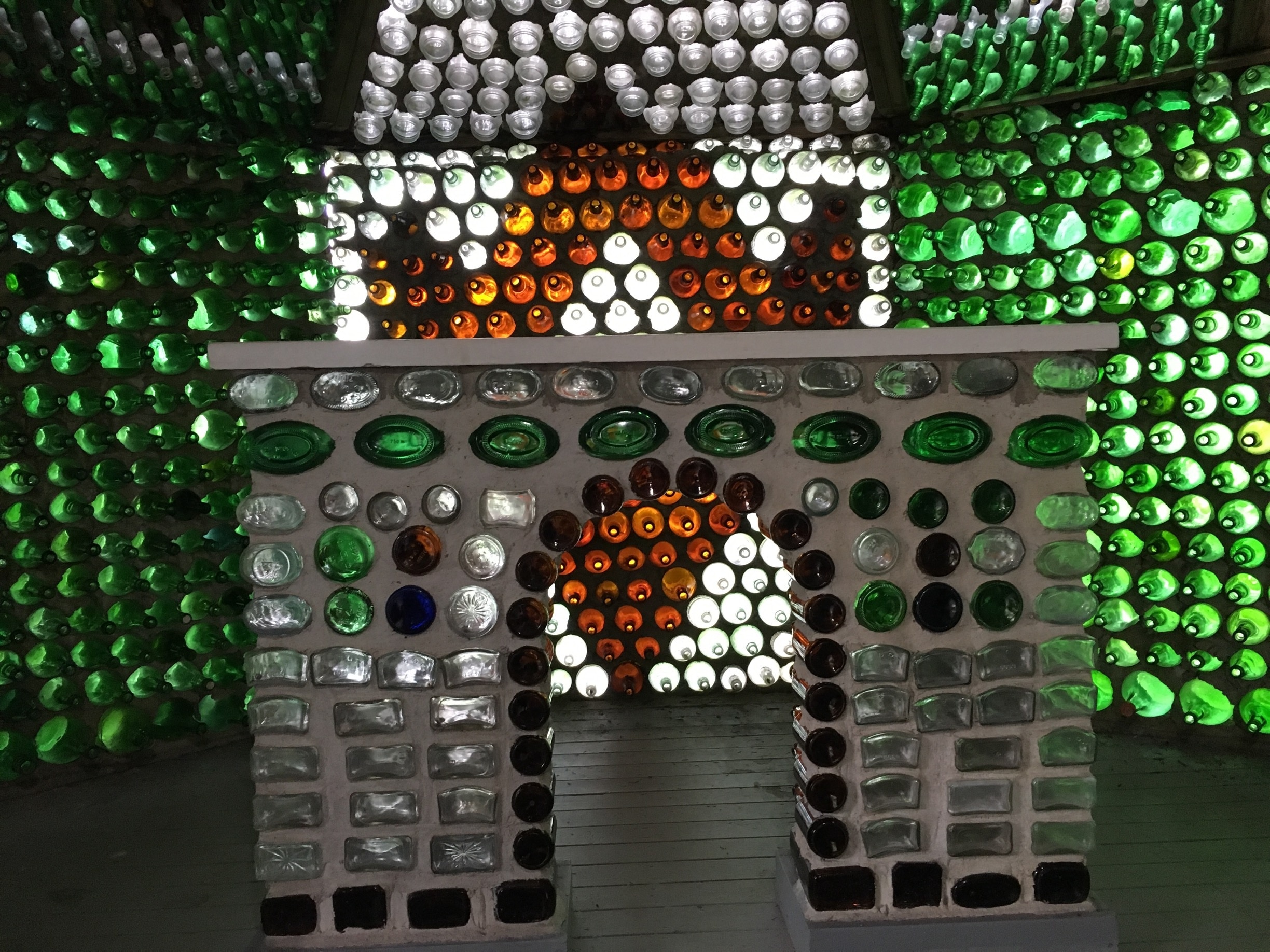The image depicts an artistic installation inside a building that closely resembles a fireplace area but without an actual fireplace. In the foreground, there is a small gateway shaped like a chimney or the front of a fireplace, constructed out of concrete. This structure is adorned with variously shaped and colored glass pieces that look like jewels, including clear, green, white, and orange bottles and panels. The bottom features rectangular glass areas while the top displays circular ones, including a row of green circular glass.

The installation sits on a gray painted wooden floor. Surrounding the fireplace-like structure are three walls embedded with numerous glass bottles. The left and right wall panels predominantly feature green bottles, while the center wall showcases a mix of white and yellow bottles. All these glass elements are backlit, causing the entire room to glow and creating intricate light reflections. Above, a reflective surface or mirror amplifies the glowing effect of the installation. Overall, the scene is a mesmerizing and vibrant representation of light and color, designed to evoke the artistic and creative essence of the space.